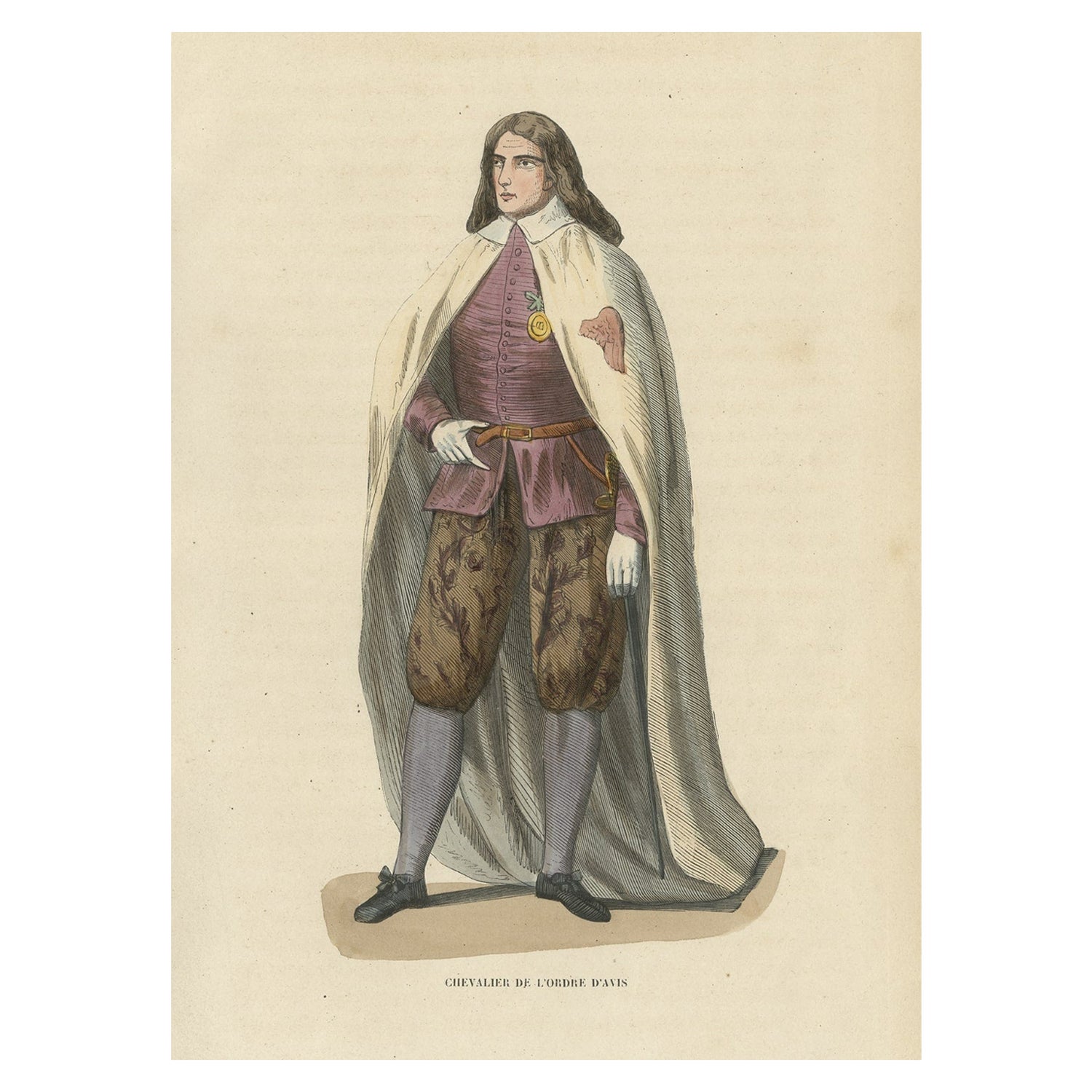The illustration depicts a high-class man from an earlier time period, rendered with meticulous detail on light brown paper. He stands in a poised manner with his right hand resting on his waist, touching a brown belt that cinches his maroon doublet. This doublet, adorned with buttons and a metal on the left chest, tops his brown pantaloons that end at the knee, transitioning into tall, bluish-gray socks and black shoes. Over his attire, he wears a long, flowing pale-colored cloak with a white collar, featuring a distinct maroon cross on the left side. His long, silky brown hair cascades past his shoulders, framing a clean-shaven face with long eyebrows. The background of the drawing has an antique beige tint, and at the bottom, the caption in black uppercase letters reads "Chevalier de Lougeray-Davy."